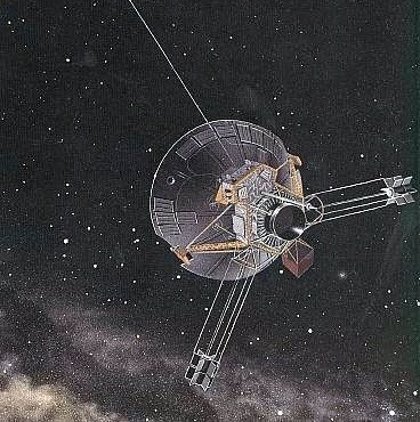This detailed image, likely an artist's rendering, depicts a satellite floating in the vastness of space. The primary backdrop is a black sky scattered with speckles of white representing distant stars. In the bottom left corner, there are gray and white light clouds, adding a touch of cosmic ethereality. Centered in the image, the satellite itself is the focal point. It's predominantly circular, with a gray dish and an attached black circle at its back. A small brown box is situated beneath this black circle. Extending from the dish are several thin rods or antennas; one is directing toward the top left, and others fan out to the right and bottom left. The color palette of the image includes black, white, gray, silver, gold, yellow, and maroon, which contribute to its realistic yet artistic appearance. The overall scene exudes a sci-fi feel, emphasizing the satellite's presence amidst the stars and stellar clouds, marking its place in the deep expanse of space.